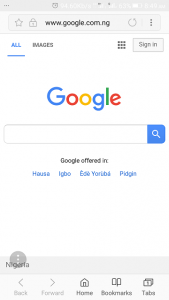The smartphone screen displays several icons and interfaces, including a holographic star icon, a lock icon, and a web address bar showing "www.google.com.ng." There are buttons for refreshing the page and a "more options" button represented by three vertical dots. The screen predominantly shows a Google Images search page with a blue header, which reads "All Images." A numeric string "124689" appears, indicating a possible search result count or identifier. The page also includes a "Sign In" prompt and prominently features the Google logo, with the blue colored letter "G" followed by alternating letters "o" in blue and red.